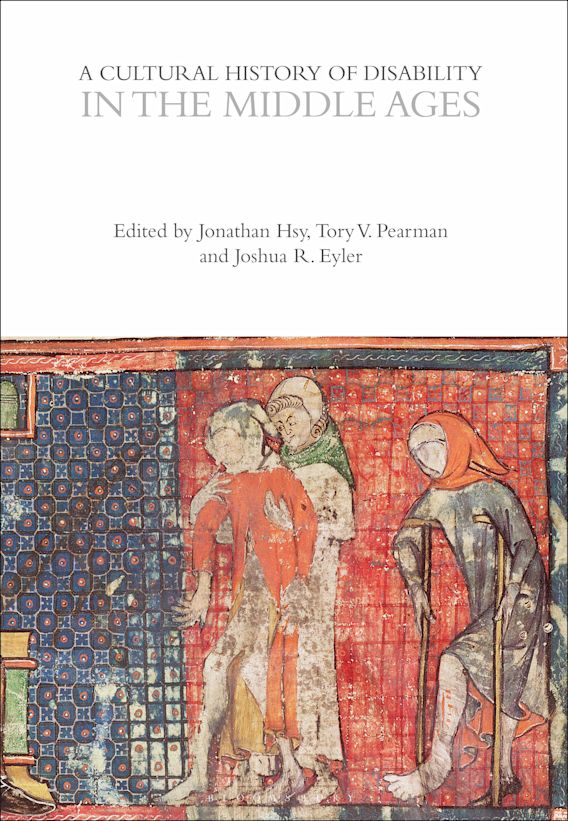The image depicts the cover of a book titled "A Cultural History of Disability in the Middle Ages," edited by Jonathan Tsai, Tori V. Pearman, and Joshua R. Eiler. The title is prominently displayed in bold letters at the top center, followed by the editors' names in smaller print. Below this text, the book cover features an intricate mosaic-like painting that dominates the bottom half of the cover. The painting, rendered primarily in red hues, portrays three individuals. 

The first person, appearing distressed, is dressed in a reddish robe and is being supported under the armpits by a second figure. This second person, who is possibly a woman, wears a green scarf along with a bonnet. Behind them, slightly more to the right, stands a third individual on crutches, dressed in a gray robe and an orange bonnet, noticeably barefoot. To the left of this scene, the mosaic transitions into a section with blue tiles, adding contrast to the red-centric background. The entire image evokes an ancient, rustic feel, reminiscent of historical paintings or murals, suggesting a scene from a long-gone era reflecting themes of disability and support.